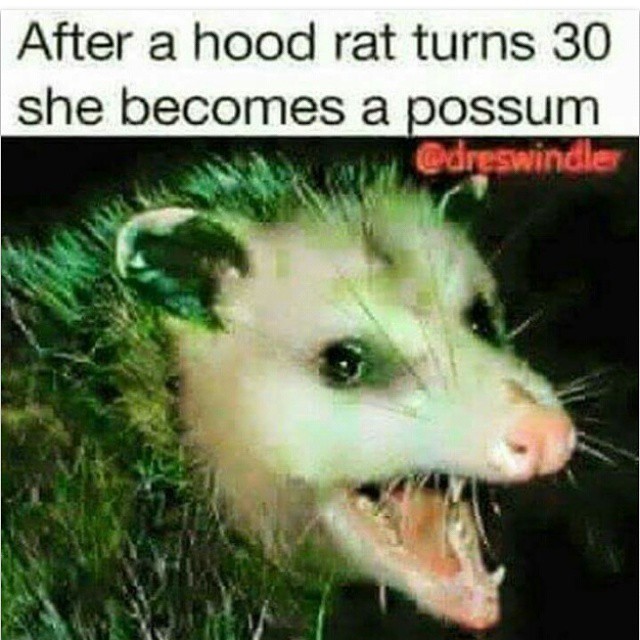The image is a meme poster with a black background featuring a close-up, slightly low-resolution photograph of an opossum's face. The opossum, primarily white with black-tipped ears and spiky fur, has its mouth open as if it is screaming, showing its sharp teeth, light pink nose, and tongue. Its head is turned slightly to its left, making it appear as though it is looking directly at the camera. Above the opossum, black text on a white background reads, "After a hood rat turns 30, she becomes a possum." In the top right corner of the photo, red text reads, "@DrezSwindler." The image has been compressed, causing some blotchy artifacts. Overall, the meme conveys a satirical and humorous message, often shared on social media.